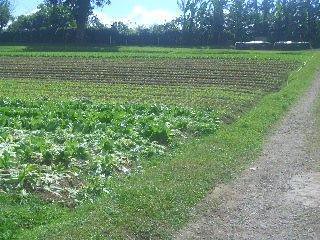The image depicts a well-organized farmer's field. The foreground features rows of planted vegetation, likely leafy greens such as lettuce. These rows are bordered by patches of green grass and areas of brown dirt, suggesting a mix of cultivated and uncultivated sections. To the right, a gravel road, reminiscent of an unpaved driveway, winds from the front to the back, interrupted by a light patch of gravel forming a small circle. Beyond the rows of plants, a tree line stretches across the horizon, with tall trees encircling an opening that reveals a serene, powder blue, and white sky. In the distant background, there are hints of buildings nestled among the trees. A walk trail meanders along the edges of the vegetable field, highlighting the functionality and maintained order of this agricultural scene.